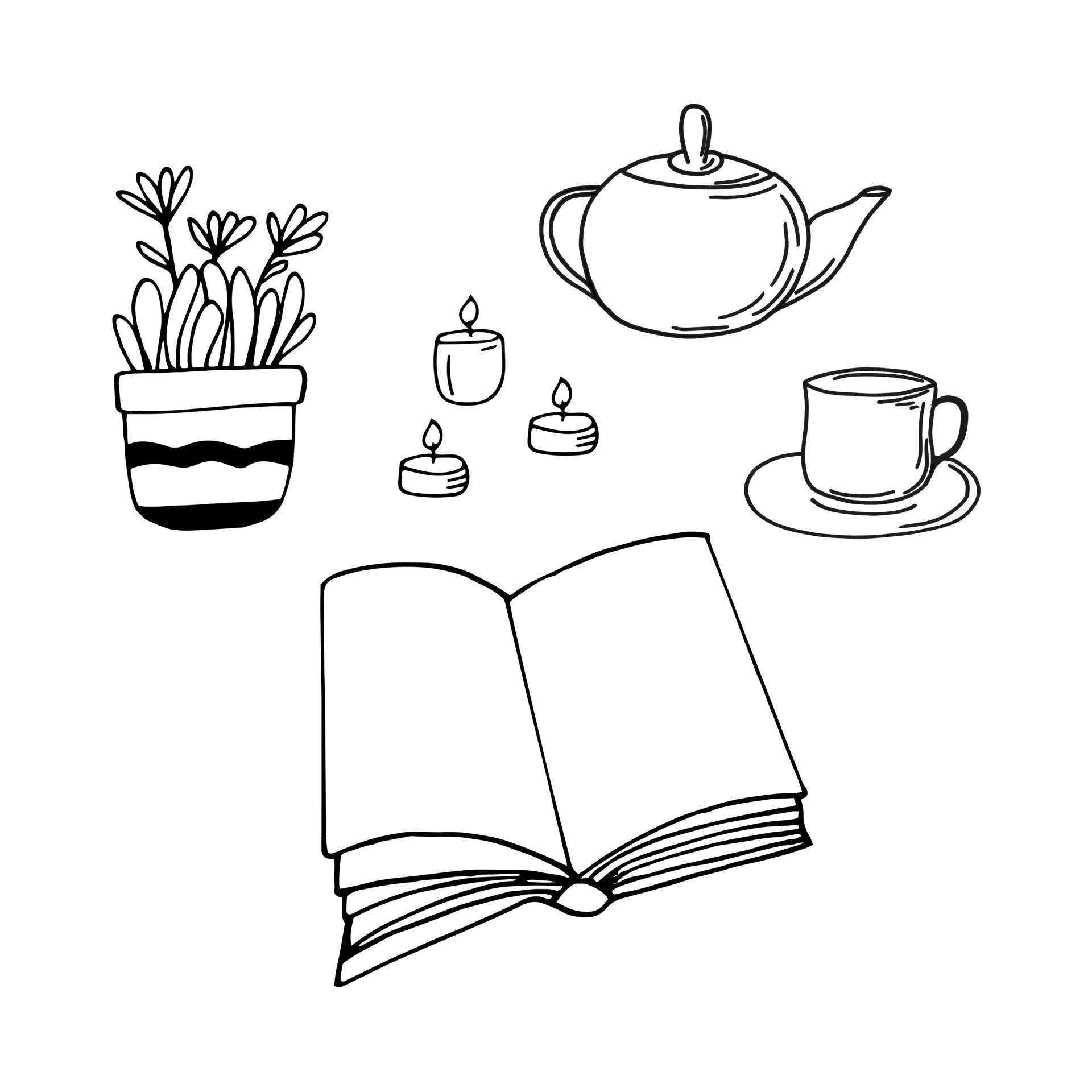This image features a series of simple, monochromatic black ink line drawings of common household items on a white background. In the upper left corner, there is a potted plant with black wavy stripes decorating the pot. The plant has a few leaves and three flowers, each with four petals, and the outer flowers also have one leaf each. At the center of the image, there are three lit tea light candles with black outlined flames. Below the candles, a blank open book is depicted, showing its middle pages. To the right of the book, there is a teacup on a saucer, and next to the teacup, in the top right corner, stands a teapot with a lid on.